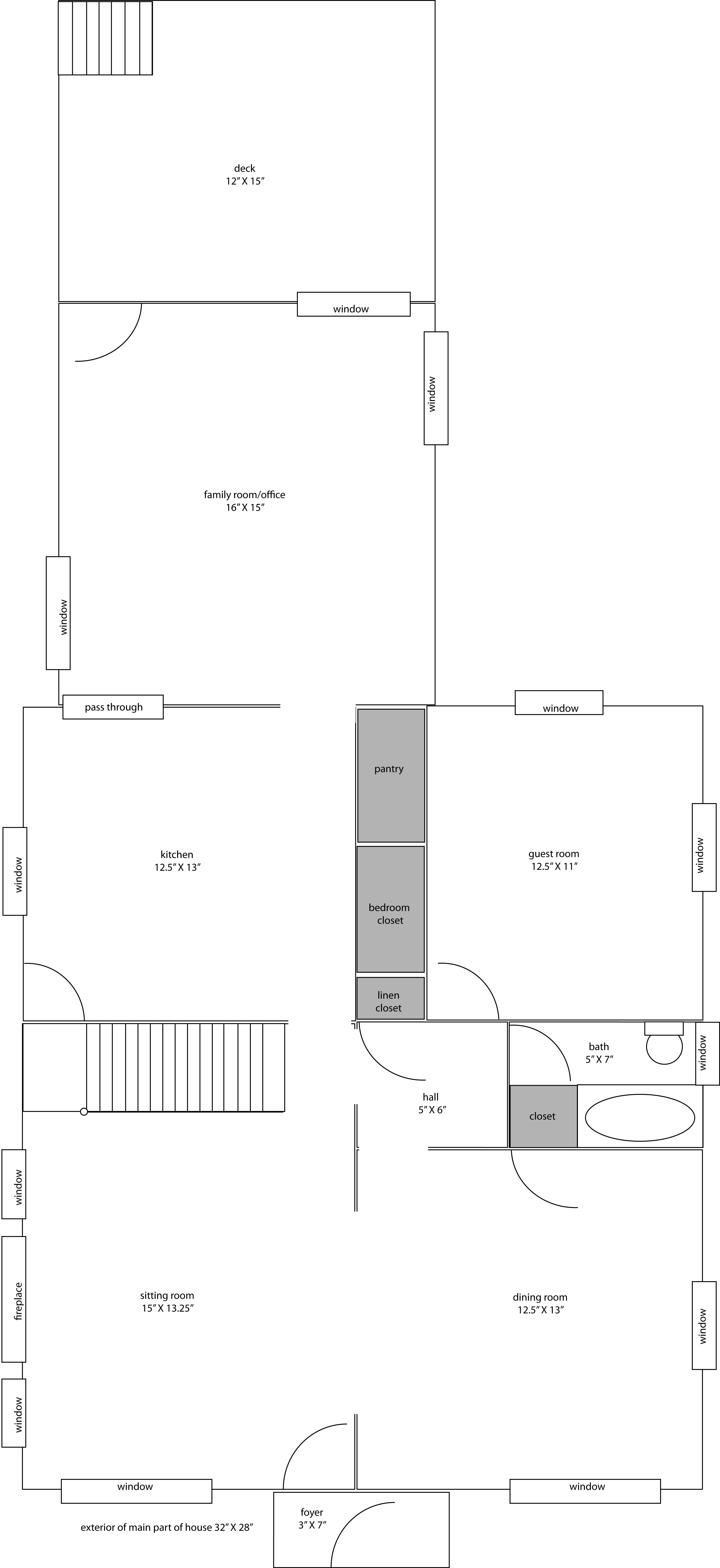This detailed floor plan illustrates the layout of a residential space, labeled "Deck 12 by 15 feet" at the top. The main sections include a multifunctional Family Room/Office, and a Kitchen measuring 15.5 by 13 feet on the bottom left. Adjacent to the Kitchen, on the right, is a Guest Room sized at 12.5 by 11 feet. Directly below the Guest Room is a Bath, with dimensions of 5 by 7 feet. 

To the left of the Bath is a Hallway, which measures 5 by 6 feet, while further to the left, occupying the bottom left corner of the floor plan, is a Sitting Room at 15 by 13 feet. On the right side of the plan is a Dining Room, which measures 4.5 by 13 feet. Below the floor plan is a compact Foyer, sized at 3 by 7 feet.

The exterior dimensions of the main part of the house are 32 by 28 feet. This layout includes several windows: one on the exterior left side, two flanking a Fireplace in the Family Room/Office, another set in the Kitchen, and a window in the Family Room/Office.

In summary, this comprehensive layout captures the spatial organization and dimensions, highlighting key areas such as the family and dining rooms, as well as window placements and additional features like the fireplace.